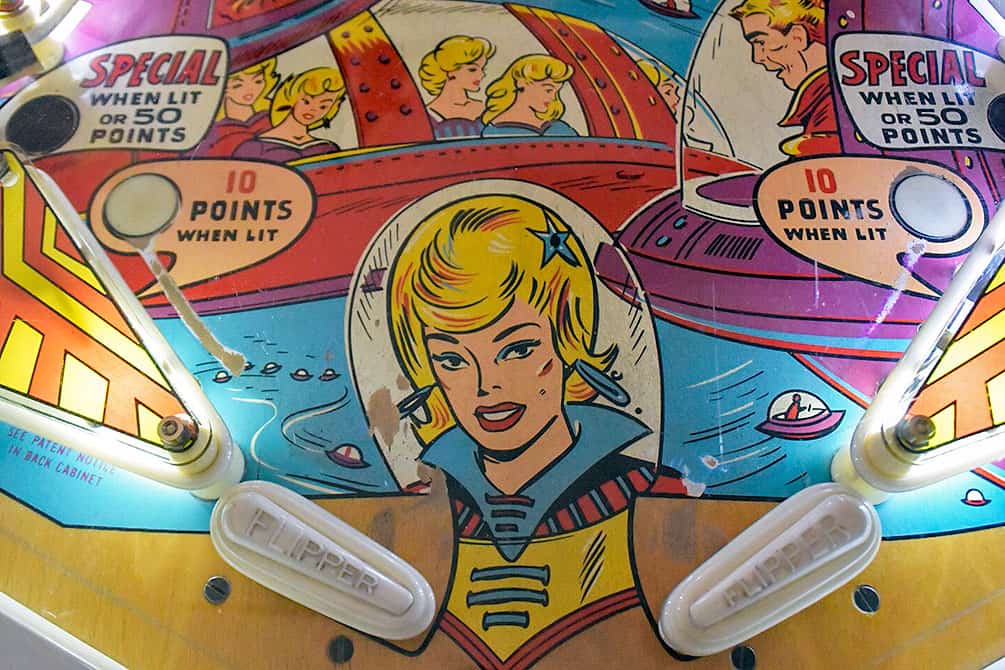The image showcases a detailed close-up photograph of the bottom section of a pinball machine's playing field. Centered at the bottom are two white plastic flippers, each engraved with the word "Flipper." Surrounding the flippers are lit white bumpers with graphic designs incorporating orange and yellow lines. Above the flippers, the playing field features an intricate comic book-style artwork. The scene includes a woman with yellow hair wearing a blue, yellow, and red top, and adorned with a star atop her head. She appears to be in a space suit, complete with a glass covering her head, emphasizing a vintage space theme. To her right, a spaceship and several other characters, including a man in another spaceship, add to the cosmic narrative. The artwork is detailed with various text bubbles that read "Special When Lit," "50 points," and "10 points when lit." Below the flippers, there's additional text stating, "See Patent Notice in Back Cabinet." The entire image captures a vibrant, retro, outer-space aesthetic central to the pinball machine's design.